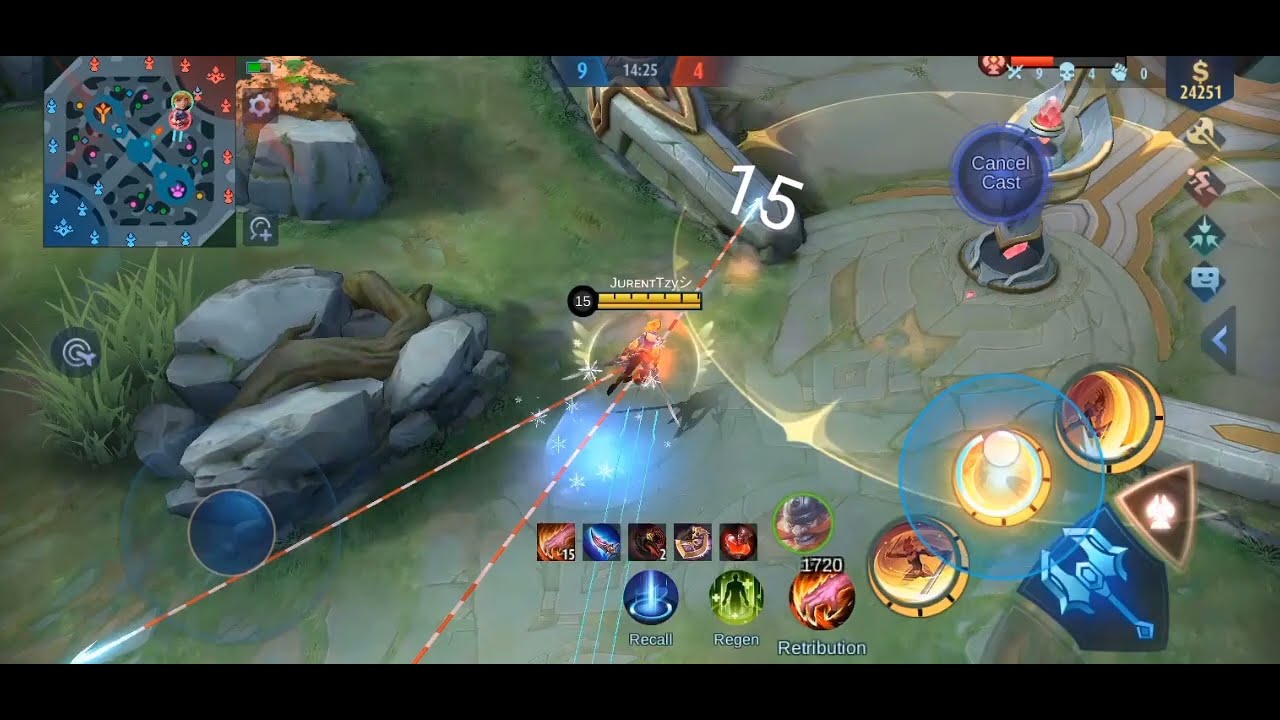This image is a detailed screenshot from a video game, viewed from a bird's eye perspective, likely captured from a mobile device or computer. The setting has a cartoonish aesthetic with a green background featuring animated rocks and grass. In the center, a character is engaged in action, possibly shooting at an enemy, with bullets visually represented by a red and white streak. A number "15" extends from the character, indicating either damage or a score.

The screen is scattered with various interactive buttons and icons. In the lower section, there are five small squares depicting different figures including a sword, a flaming fist, and a glowing symbol. Below these squares are three major action buttons: a blue one labeled "Recall," a green one labeled "Regen," and a red one labeled "Retribution" with the number 1720 above it. 

Additional elements include a mini-map in the upper left corner showing the gameplay field and more action buttons in the lower right corner, featuring icons like a blue axe, a glowing symbol, and a half-moon. The overall chaotic yet organized layout of various game elements, coupled with the numerous vibrant colors including green, gray, blue, orange, red, yellow, pink, and different shades of blue, emphasizes the dynamic and engaging nature of the game.